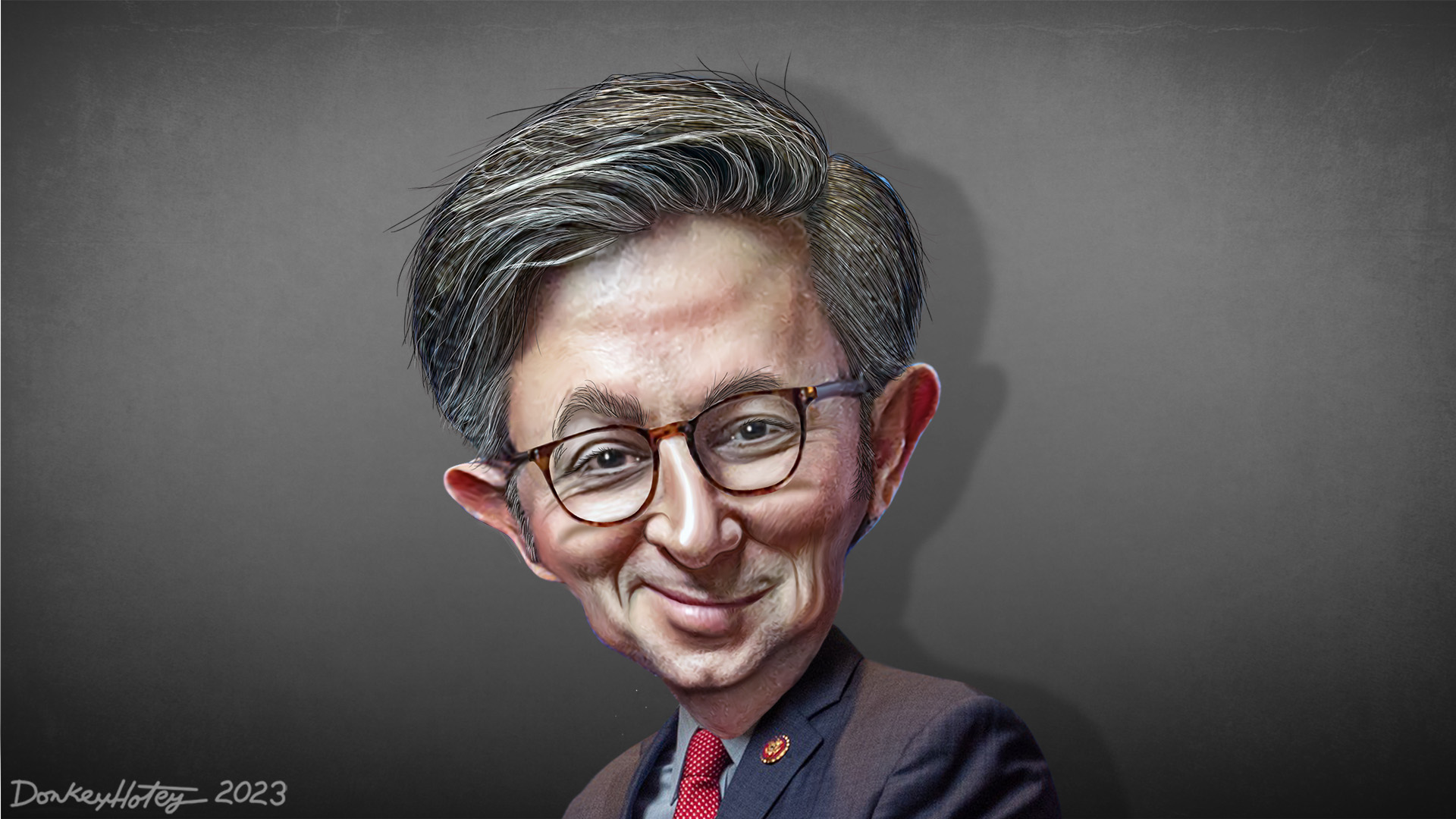This is a detailed caricature of a man, resembling a political figure, possibly the House Speaker. The cartoon shows his disproportionately large head and face, tapering from the forehead to the chin, and some part of his upper body. His gray, somewhat whitened hair is brushed to the side, and he wears brown-rimmed glasses over his brown eyes. The man's white and reddish skin is accentuated by his slightly smiling, almost smirking closed-mouth expression, looking straight at the viewer. He's dressed in a navy blue suit jacket, a light blue button-down shirt, and a red tie. The background is completely gray with a subtle black vignette effect. At the bottom left corner, there is the artist's signature, "Don Quijote, 2023."